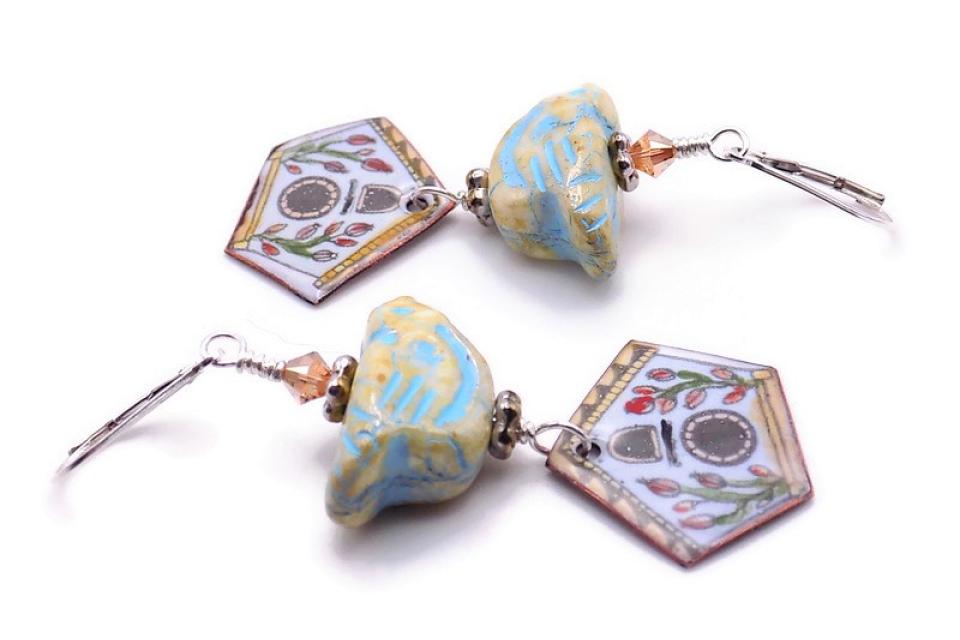The image depicts a pair of intricate earrings showcased on a white background. Both earrings are identical, highlighting their detailed, symmetrical design. Each earring features a metal loop at the top, transitioning into a circular section enveloped by silver coiling. Below the circular area, there's a sequence of components including a pinkish-brown bead followed by a flat silver bead. Continuing down, a depiction of a bird and a highly adorned birdhouse with a yellow roof, red flowers, and dual entry holes for birds are prominently displayed. The birdhouse sits atop a pentagon-shaped piece, adorned centrally with alternating black and white rings. Additional details include the presence of turquoise-colored rocks, and a blend of other beads and metallic elements featuring a floral motif with red flowers. The earrings cast subtle shadows, adding depth and emphasizing their three-dimensional aspects, making them appear catalog-ready.